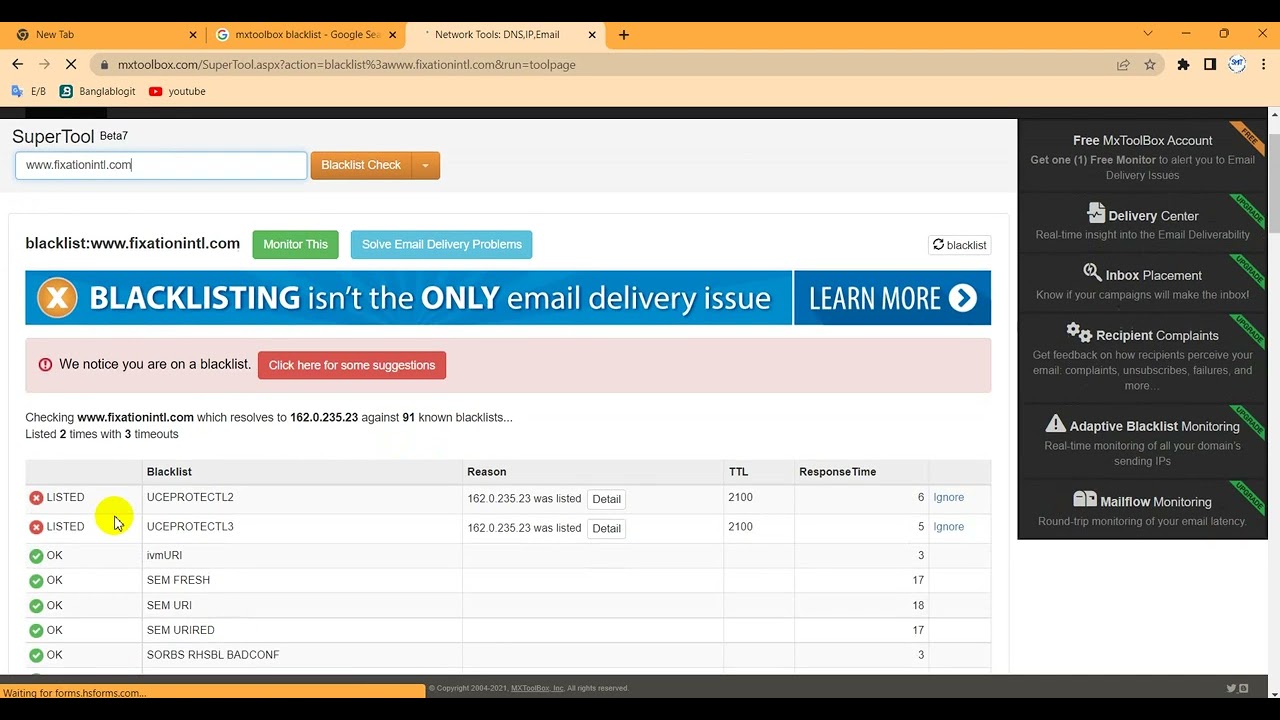This screenshot captures a website viewed on a computer, specifically showcasing MXToolbox.com's SuperTool page. Along the top of the browser are various orange tabs labeled "New Tab," "MX Toolbox," "Blacklist," "Google Search," and a peach-colored tab marked "Network Tools." Dominating the page is a prominent blue rectangle headline bar with the text, "Blacklisting isn't the only email delivery issue, learn more." Below this headline, a pink rectangle indicates, "We notice you are on a blacklist, click here for some suggestions." The content beneath this notification presents a detailed list of blacklists that the user has been flagged on. At the very bottom, there is a small orange rectangle with text that is difficult to discern due to its tiny size.